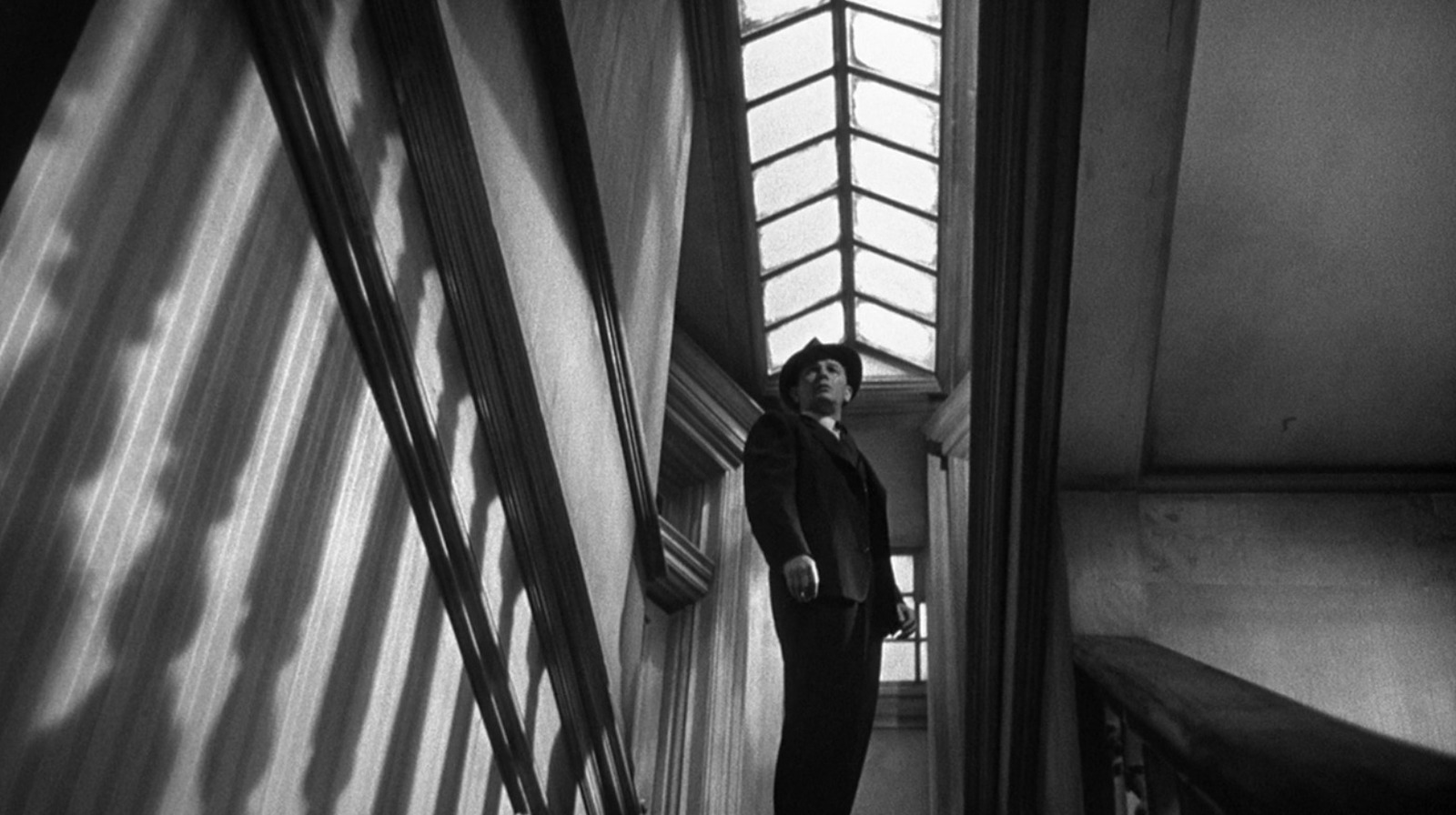The image is a striking, black-and-white photograph reminiscent of a 1940s or 1950s film still. It features a man standing in the center, dressed in a black suit and a classic fedora hat, evoking the style of a private investigator or a figure like Frank Sinatra from that era. The shot is taken from a low angle, enhancing the dramatic effect and emphasizing the architectural grandeur of the setting. The man stands motionless at the top of a staircase, surrounded by intricate, shadow-cast banisters and moldings, with light streaming in through a skylight and additional windows behind him. The overall composition, marked by dramatic shadows and elegant detailing, lends the image an artistic, almost cinematic quality, immersing the viewer in a bygone era.